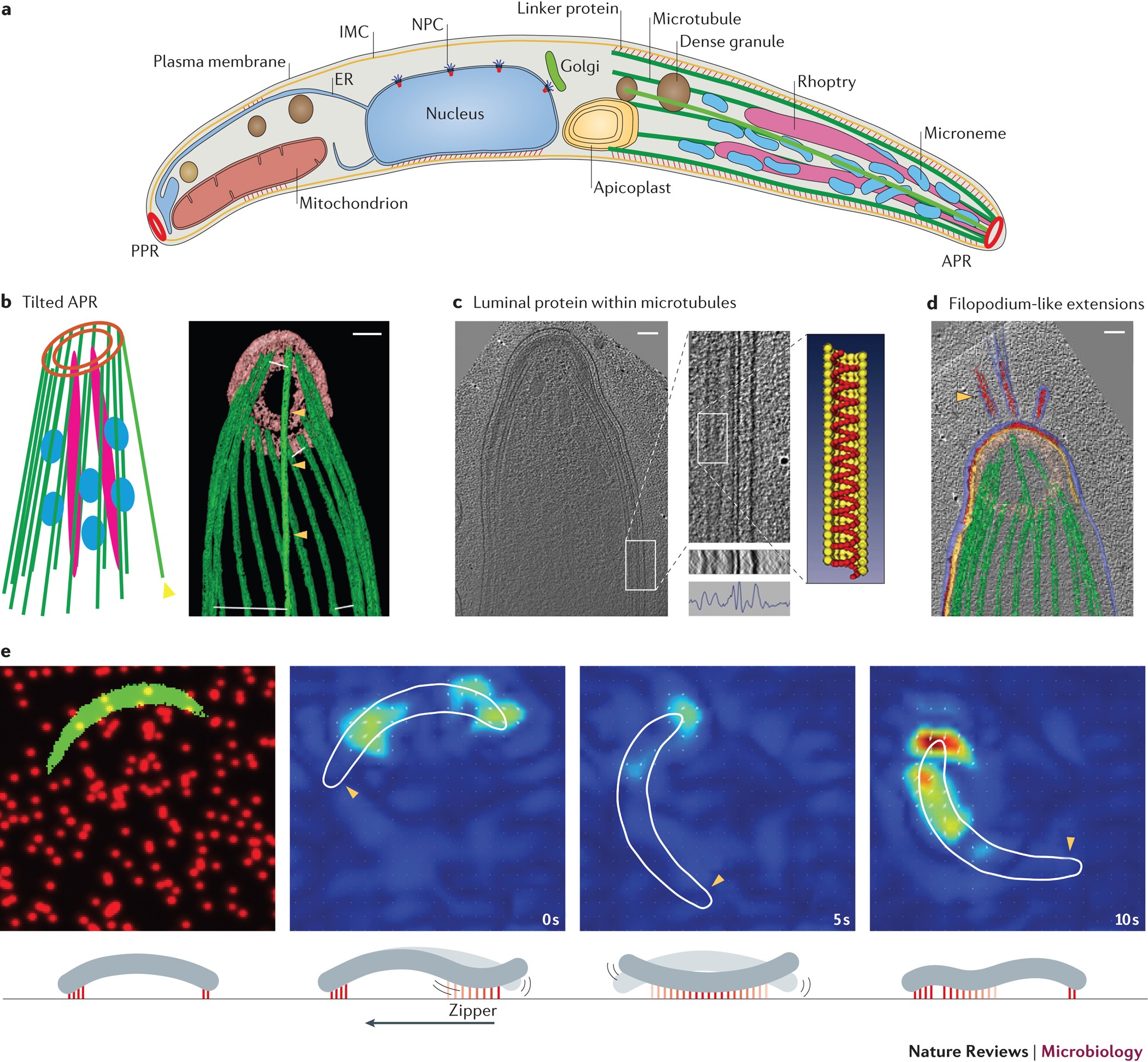This detailed scientific diagram, possibly from the microbiology section of Nature Reviews, focuses on the complex structure and dynamics of microtubules. The main image provides a comprehensive cross section, meticulously labeling every component including the mitochondrion, plasma membrane, nucleus, Golgi apparatus, apicoplast, and granules. Highlighting both a conceptual illustration and what microtubules actually look like under a microscope, the diagram offers a multifaceted view. Below the main image, four detailed photographs depict movement patterns, showing how microtubules exhibit a distinctive wiggly motion. These images vary in perspective, with some rendered in vibrant colors indicative of different protein markers, and others offering intricate, microscopic views, enriched with additional details that further illuminate the structural and functional complexities of microtubules.